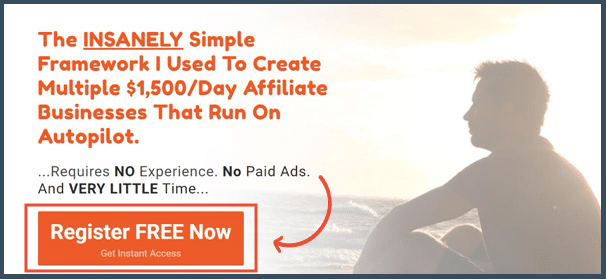The advertisement features a predominantly white background with a subtly faded, corner image of a man sitting on a beach, gazing at the waves. The primary message is conveyed in bold orange text, detailing the benefits of a tool designed for creating and managing affiliate businesses that operate on autopilot. Supplementary information, presented in dark text, further elaborates on the advantages of this app. Prominently highlighted in a large orange section, white text urges viewers to "Register for Free Now," with a smaller white text below offering "Get Instant Access."